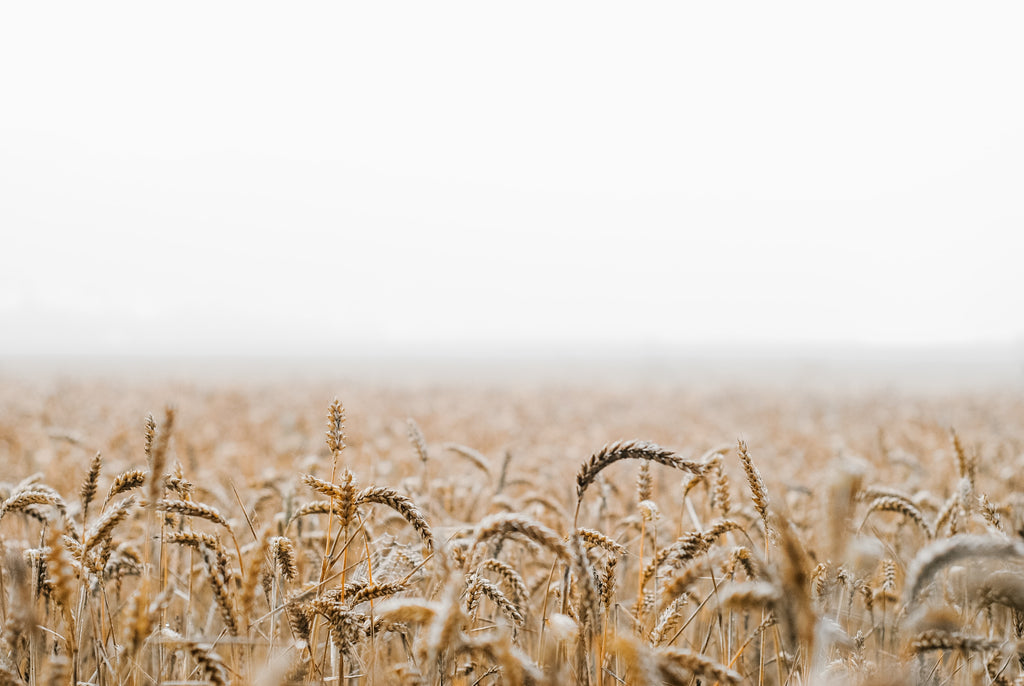This image captures an expansive field of wheat that stretches endlessly across the frame. The foreground showcases intricate details of the wheat stalks, with their heads of grain vividly rendered in varying neutral hues of beige, golden-brown, and occasional grayish tones. As the field extends into the mid-ground, the clarity diminishes, and the stalks become progressively blurry, indicating depth and distance. The serene and peaceful atmosphere is accentuated by the sky, which dominates the top half of the picture with a hazy whiteness, suggestive of an overcast or foggy day. The horizon, where the wheat field meets the sky, splits the photograph right at the center, emphasizing the vastness of the landscape and the indistinct blur of the background. This haziness creates a sense of endlessness and tranquility, making it hard to distinguish where the land ends and the sky begins. The overall composition highlights a peaceful morning in an endless wheat field, with the blurred and cloudy sky adding to the dreamlike quality of the scene.